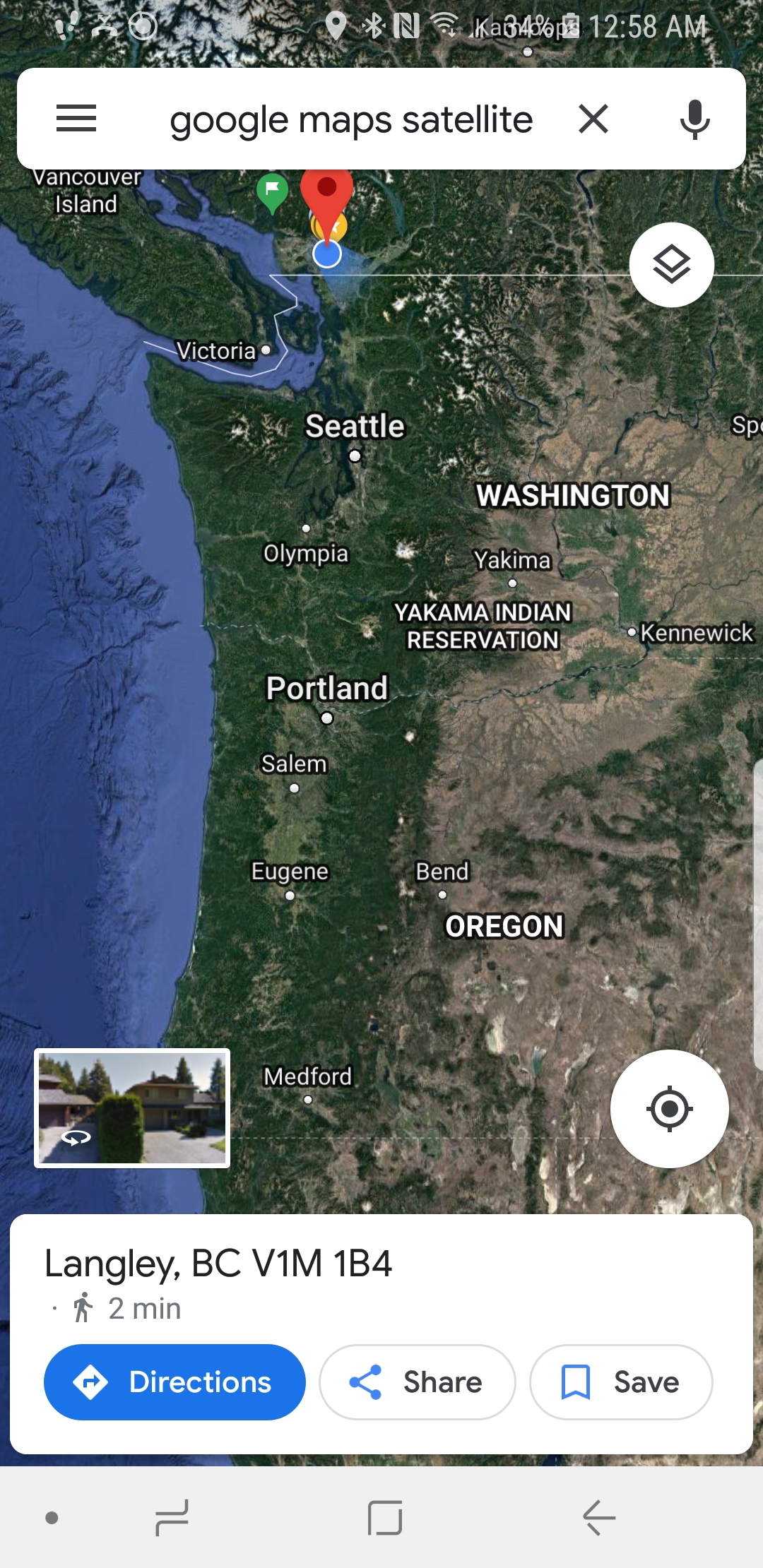The image is a detailed screenshot from a cell phone displaying a Google Maps Satellite view in portrait mode. At the top of the screen, cell phone icons such as a battery indicator at 34% and the time at 12:58 AM are visible. The search bar reads "Google Maps Satellite" and includes an 'X' and a microphone icon. The primary map display showcases an extensive overhead view of land and water, focusing on the western coast of the United States, particularly the state of Washington and Oregon. Key locations like Vancouver Island, Victoria, Seattle, Olympia, Yakima, Yakima Indian Reservation, Kennewick, Portland, Salem, Eugene, Bend, and Medford are marked. In the center of the image, some cities, notably Portland and Seattle, are highlighted in a larger font. The map also features labels for the states of Oregon and Washington. Along the right border of the map, a water body extends from the bottom to the top of the screen. At the bottom, details such as "Langley, BC V1M 1B4", a walking icon labeled "2 minutes", and options including "Directions", "Share", and "Save" are displayed, indicating walking directions in Langley, British Columbia.